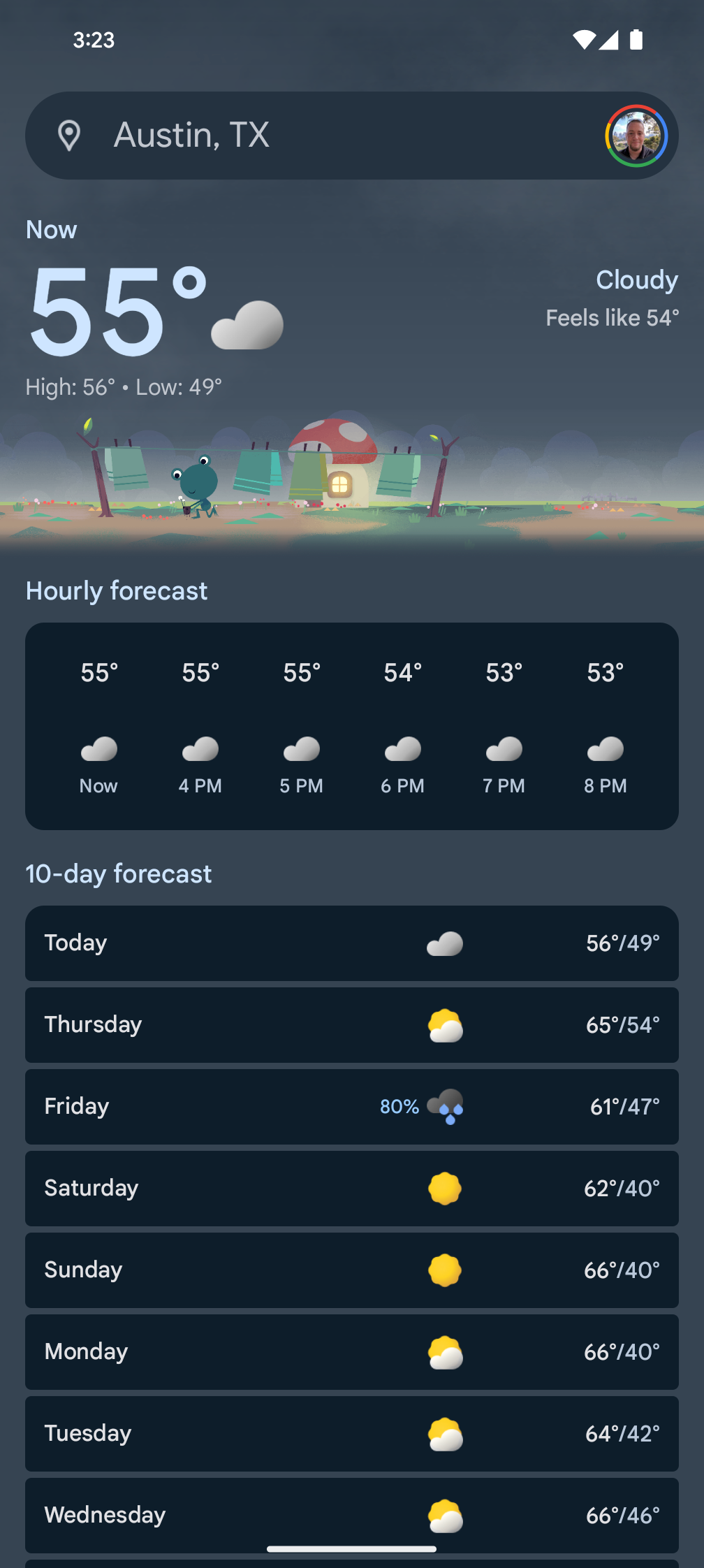The image showcases a screenshot from a weather app for Austin, Texas. In the top left corner, the current time is 3:23. Below the search bar, the present temperature is 55°F, featuring a high of 56°F and a low of 49°F. The right side indicates that it is currently cloudy and feels like 54°F. A whimsical illustration below depicts a frog hanging up towels on a clothesline outside a mushroom house. The app then provides an hourly forecast: 55°F at 3 p.m., 55°F at 4 p.m., 55°F at 5 p.m., 54°F at 6 p.m., 53°F at 7 p.m., and 53°F at 8 p.m. The 10-day forecast shows temperatures for each day, starting with today at 56°F/49°F, followed by Thursday at 65°F/54°F, Friday at 61°F/47°F, Saturday at 62°F/40°F, Sunday at 66°F/40°F, Monday at 66°F/40°F, Tuesday at 64°F/42°F, and Wednesday at 66°F/46°F.